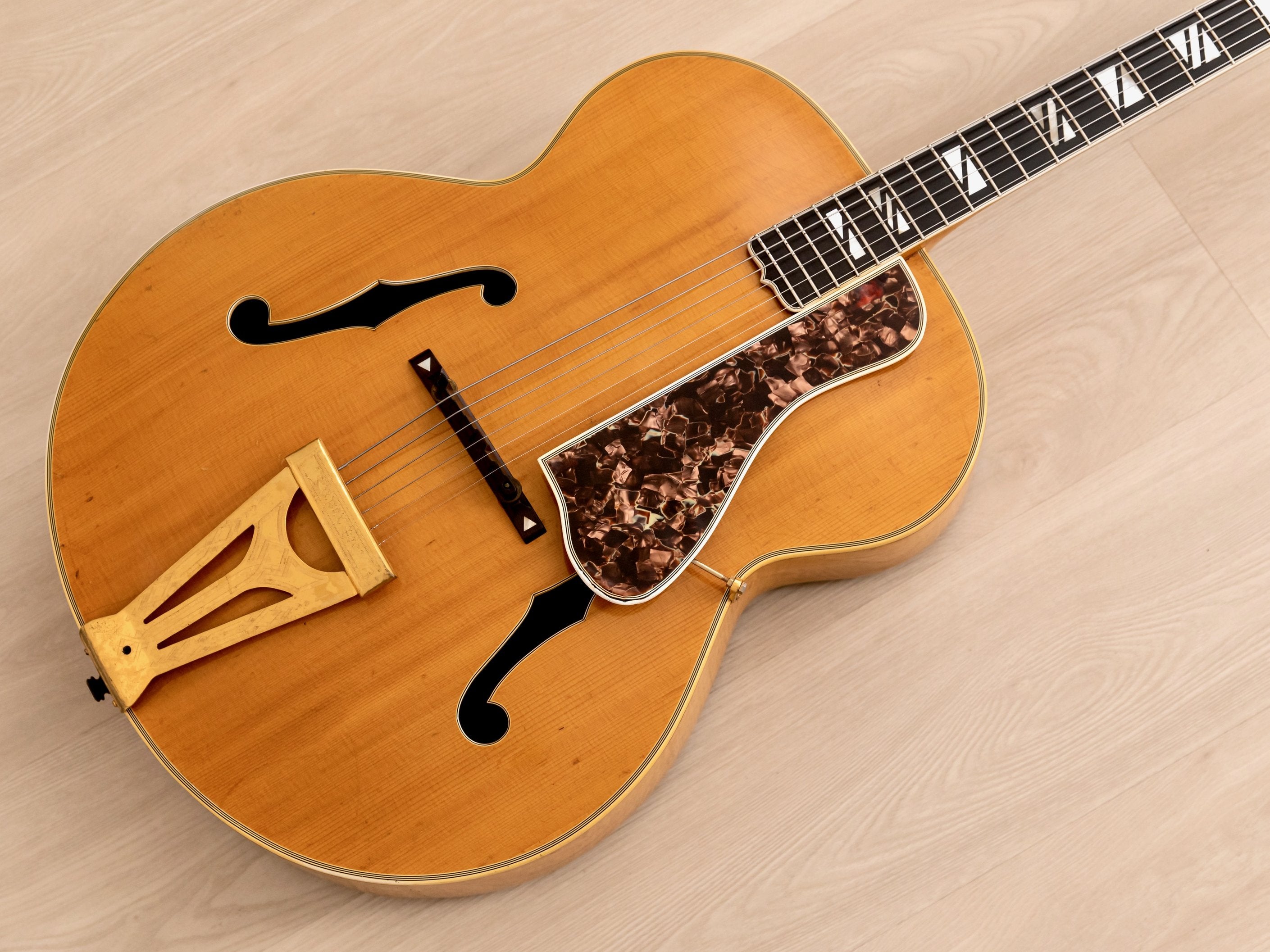This photograph, likely taken indoors, features a beautifully designed Gibson Super 400 acoustic guitar prominently displayed on a light tan synthetic wooden floor. The guitar, crafted from a golden-hued light wood, boasts a classic, slightly aged look but remains in excellent condition, free of damage on both its body and neck. Its hollow body design aligns with acoustic jazz styles and is adorned with a brown tortoiseshell pickguard, secured by a brass screw, which is accented with white and black binding. The guitar’s neck is predominantly black, embellished with white pearl inlays, and the strings are meticulously taut and secure. Notably, the guitar's body features two elegant F-hole cutouts, reminiscent of a violin, enhancing its vintage aesthetic. The intricate detail of this well-preserved instrument suggests it is a cherished piece, conveying both the artistry of its craftsmanship and its lasting musical legacy.